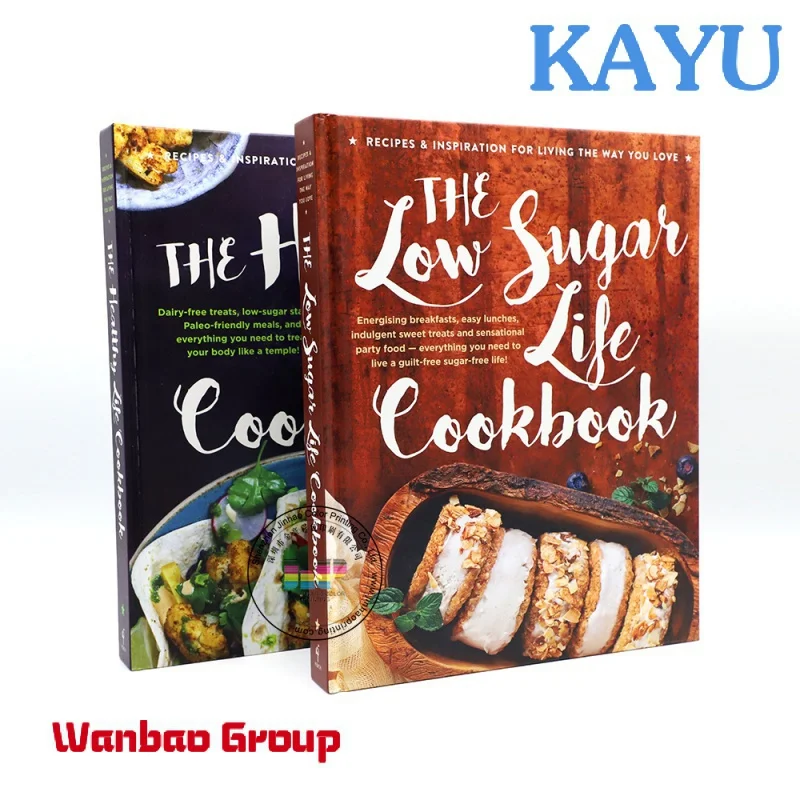The image is a photograph of two staggered cookbooks against a white background. The cookbook in the foreground has a dark orange or brick red cover and is titled "The Low Sugar Life Cookbook" in large, white, mostly cursive text. The cover features a wooden basket at the bottom filled with five ice cream sandwiches made with cookies. There is a tagline in white text across the top that reads "Inspiration for living the way you love," along with a smaller tagline to the left of the word "life," which promotes "energizing breakfast, easy lunches, indulgent sweet treats, and sensational party food for a guilt-free, sugar-free life." The second cookbook, partially obscured behind the first, has a black cover with text that emphasizes "Dairy-Free Treats, Low Sugar, Paleo-Friendly Meals, everything you need to treat your body like a temple." The cover appears to show a dish that includes a flour tortilla with meat and green leaves, possibly spinach. There is text in blue on the upper right corner of the photograph that reads "Caillou," and red text on the lower left that says "Wanbao Group."